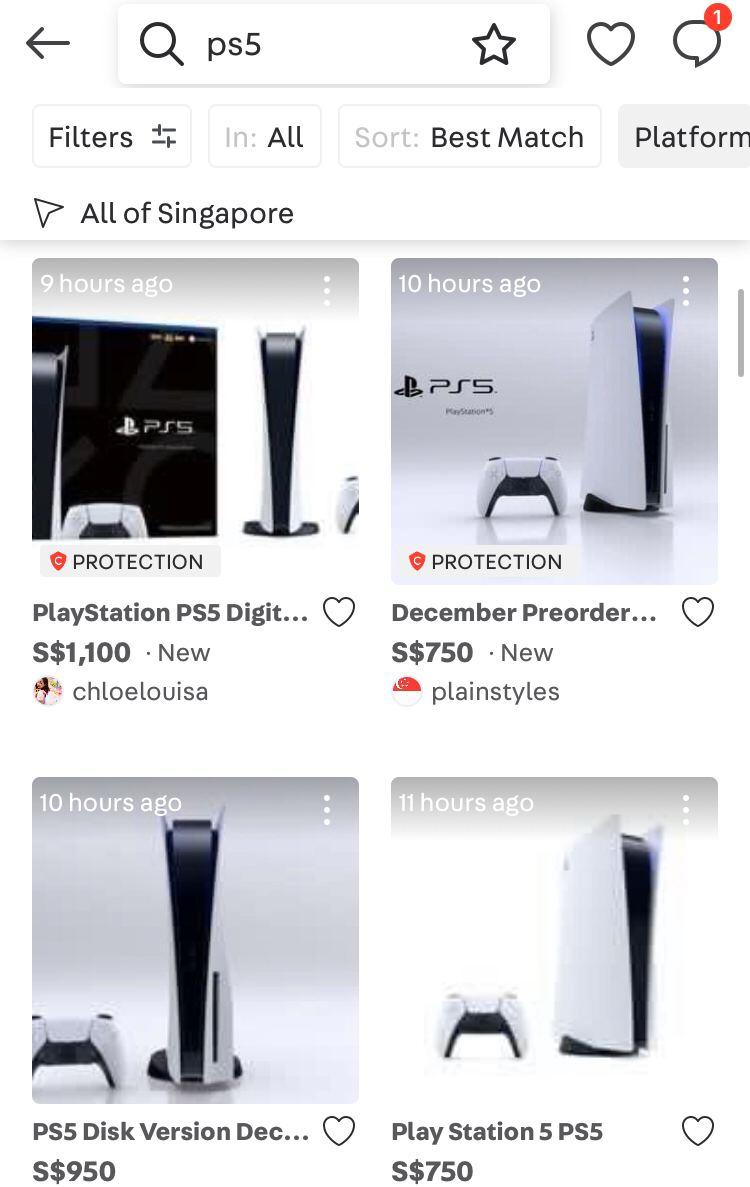Screenshot from an Online Marketplace Showing PlayStation 5 Listings in Singapore

The image is a screenshot from an online marketplace showing the search results for "PlayStation 5" in Singapore. It includes various UI elements like filters and a sort option set to "Best Match." The geographic filter is set to "All of Singapore."

The results show four listings, all posted approximately nine to ten hours ago. Here are the details of each listing:

1. **PlayStation 5 Digital Edition**
   - **Price:** $1,100
   - **Seller:** Chloe Luisa
   - **Time Listed:** 9 hours ago
   - **Protection:** Yes

2. **PlayStation 5 December Pre-order**
   - **Price:** $750
   - **Condition:** New
   - **Seller:** PlainStyles
   - **Time Listed:** 10 hours ago
   - **Protection:** Yes
   - **Description:** White PS5 model
   
3. **PlayStation 5 Disc Version**
   - **Price:** $950
   - **Time Listed:** 10 hours ago
   - **Protection:** Not specified

4. **PlayStation 5 (1TB)**
   - **Incomplete Description:** The listing mentions "10" which might be a typo or abbreviation. Possibly 1TB.
   - **Price:** Not clearly specified
   - **Time Listed:** 10 hours ago
   - **Protection:** Not specified

Protection status is available for the first two listings, while the latter two do not specify protection and the seller information for these listings is not visible.